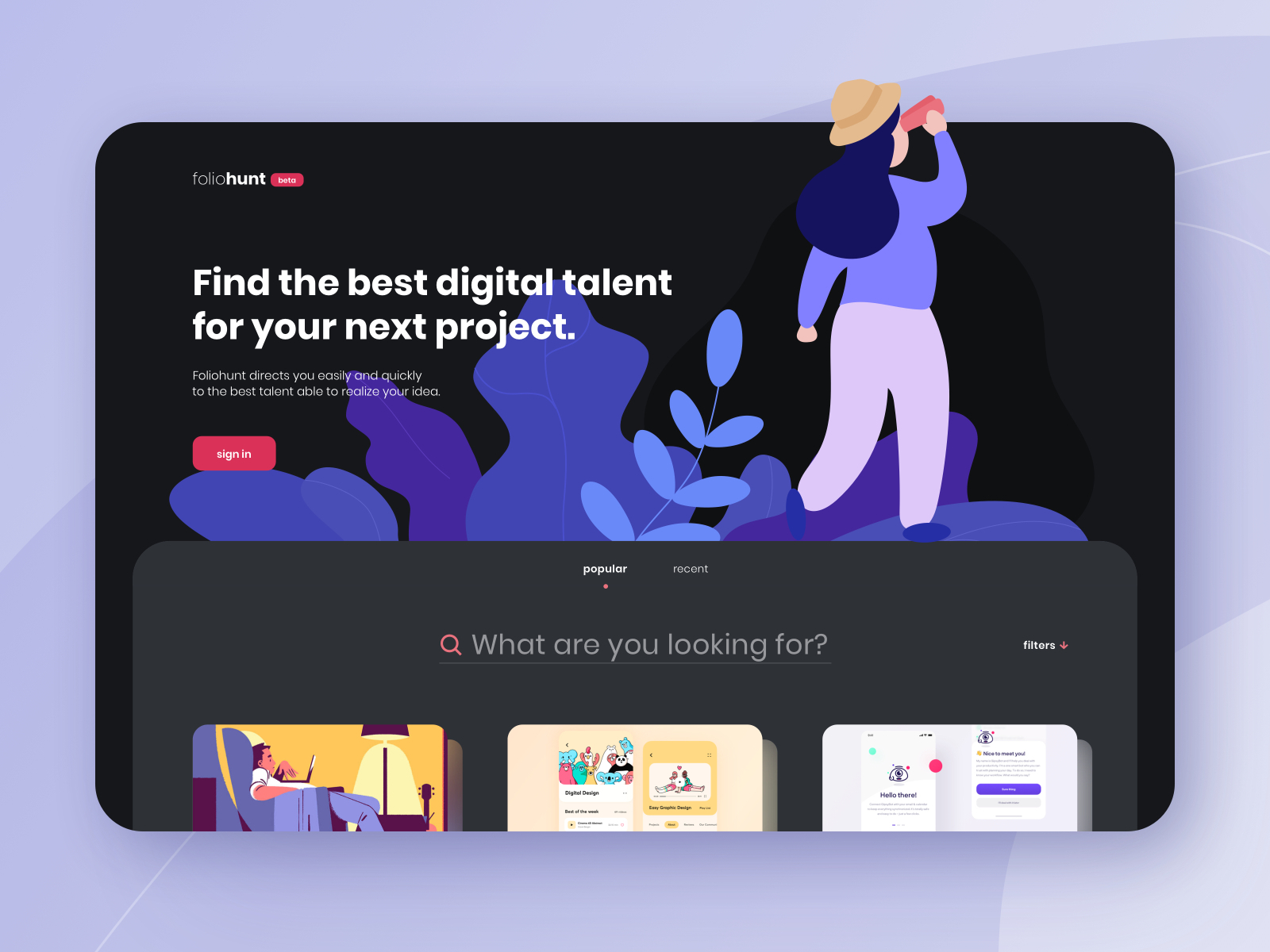Here's the cleaned-up and detailed caption for the image:

---

This image is a screenshot of a website called Folio Hunt. The website's header, located at the top left, displays the name "Folio Hunt" prominently. Directly beneath that, there is a tagline that reads, "Find the best digital talent for your next project," further emphasized by a smaller text description below, "Folio Hunt directs you easily and quickly to the best talent able to realize your idea." 

A red "Sign-In" button is positioned below this text. To the right of the text, there is a vibrant graphic featuring a woman. She is depicted looking upward through red binoculars, donning a purple sweater, dark blue hair, gray pants, and an explorer hat, suggesting she is searching for talent. The background around her implies she's in a forest, reinforcing the theme of searching or exploration.

Below this, there are two tabs: "Popular" on the left and "Recent" on the right. The "Popular" tab is currently selected. Under these tabs lies a search bar prompting users with the question, "What are you looking for?" Users can type their queries directly into this search bar.

Further down, the layout includes three image thumbnails. The leftmost image features people sitting down, while the two images to the right display various web pages.